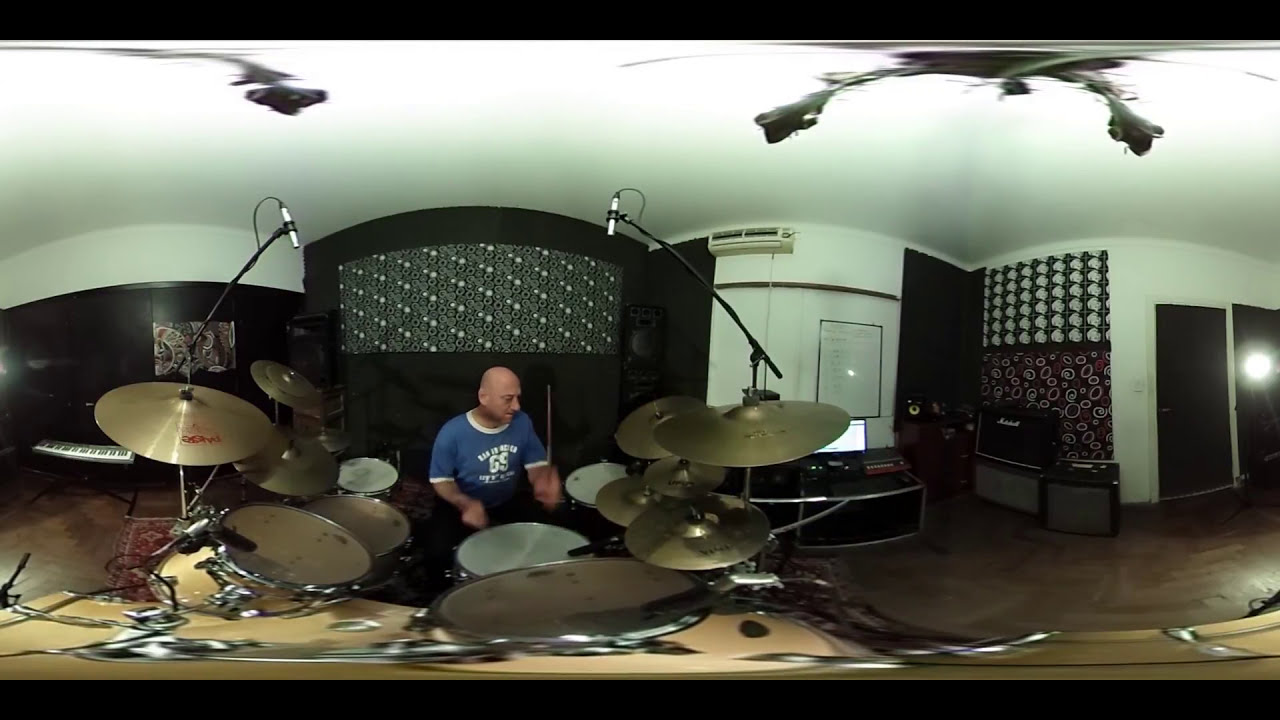This panoramic photograph captures a bald man, likely in his 40s or 50s, fervently playing a large drum set. The man, positioned centrally and visible from the waist up, is dressed in a dark blue short-sleeved shirt adorned with white stripes on the sleeves and neckline, though the text on his shirt is unreadable. His caramel-colored skin adds a rich contrast to the vibrant hues of his attire.

The drum set is extensive, featuring numerous drums and cymbals, indicative of his experience and dedication as a drummer. The man's dynamic pose shows one drumstick hitting the drum while the other is raised midair, emphasizing the action of his performance. Overhead microphones hang, suggesting this might be a recording session to amplify and capture the intricate sounds of his drumming.

The room is spacious with white-painted walls, a ceiling fan at its center, and a white ceiling. A mounted air conditioning unit is present on one wall, ensuring a comfortable environment. On the right side of the image, dark brown wood flooring and a white-framed two-pane glass sliding door add to the room's aesthetic. A plastic light switch and various speakers and subwoofers are noticeable, with additional musical equipment like a keyboard seen nearby, reinforcing the sense that this could be a professional recording or practice space. The setting is neat, albeit filled with the necessary equipment for a dedicated musician.